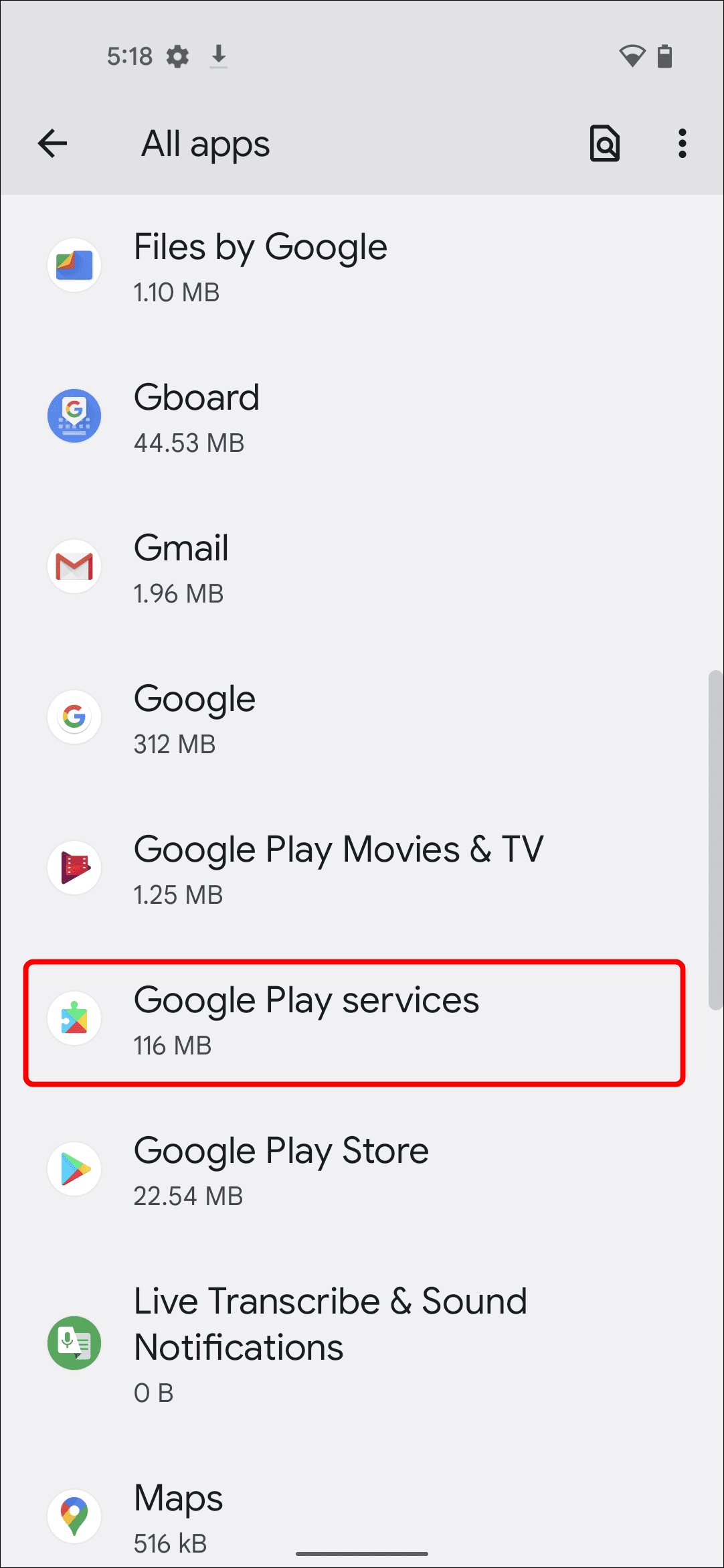The image shows a screenshot from a smartphone, specifically focusing on the "All Apps" section within the settings menu. Each app is listed with its corresponding storage size in megabytes. 

Highlighted with a red box is "Google Play services," which occupies 116 MB. The other apps and their sizes displayed in the list include:
- Files by Google: 1.1 MB
- Gboard (Gboard): 44.53 MB
- Gmail: 1.96 MB
- Google: 312 MB
- Google Play: 1.25 MB
- Google Play Store: 22.5 MB
- Live Transcribe: 0 bytes (anomaly noted by the observer)
- Maps: 516 MB

The icons for each app are vividly colored, such as the Google Play icon featuring a blue, red, and orange triangle. The background of the app list is predominantly black, with the names and sizes of the apps in white text. 

At the top of the screen, the header bar is a darker shade of gray, providing access to app-related actions such as a document search icon and a three-dot menu for additional settings. This detailed view of the "All Apps" section reveals the storage usage of various Google apps on the smartphone.